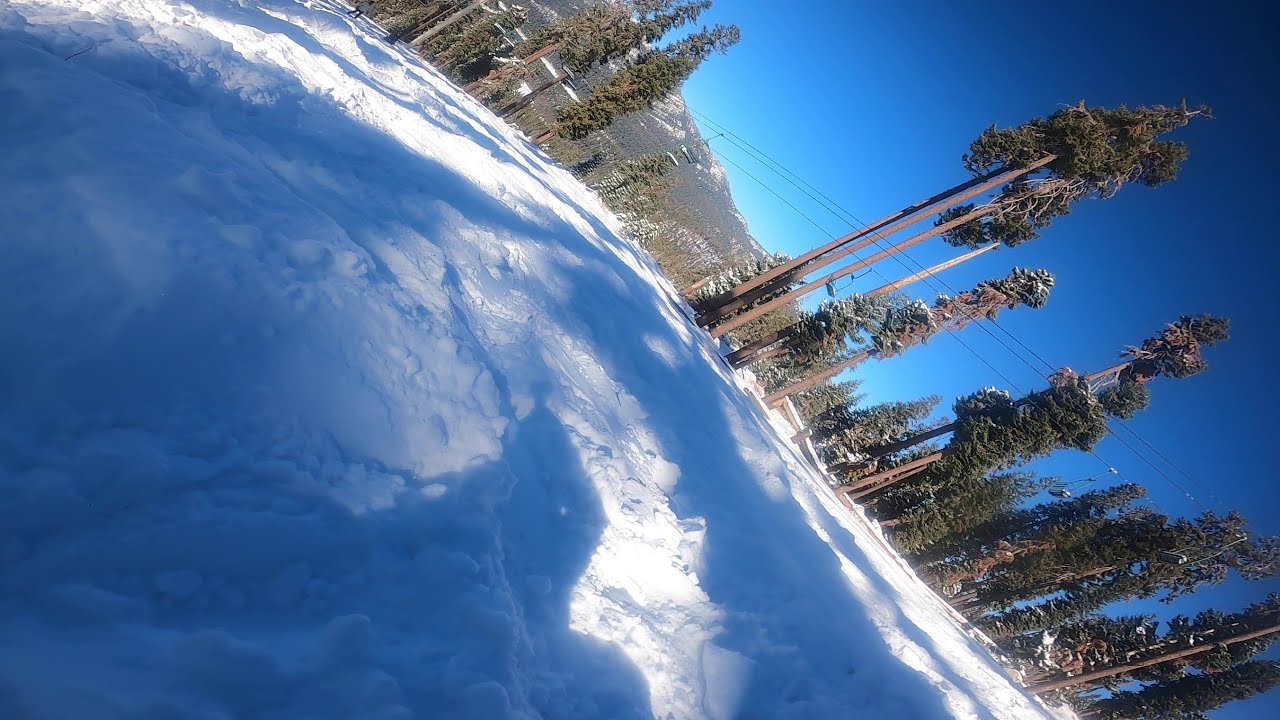The image presents a unique and slightly disorienting outdoor scene dominated by snow, trees, and distant mountains, with a noticeable tilt of about 45 degrees to the right. The snow-covered landscape features rough, powdery textures with grooves, paths, and a mixture of large and small snow chunks spread across the field. Dark shadows are cast over the snow from tall, thin trees that line the horizon. These trees have bare trunks with foliage mostly concentrated at the tops and seem to stretch diagonally from the bottom right to the top left corner. Beyond these trees, you can glimpse a range of prioner spruce trees and rocky, earthy-colored mountains. In the background, the sky transitions from a dark, cerulean blue on the right edge to a brighter blue towards the center, enhancing the serene and shadowy atmosphere. Additionally, telephone lines are visible cutting across the scene above the trees.